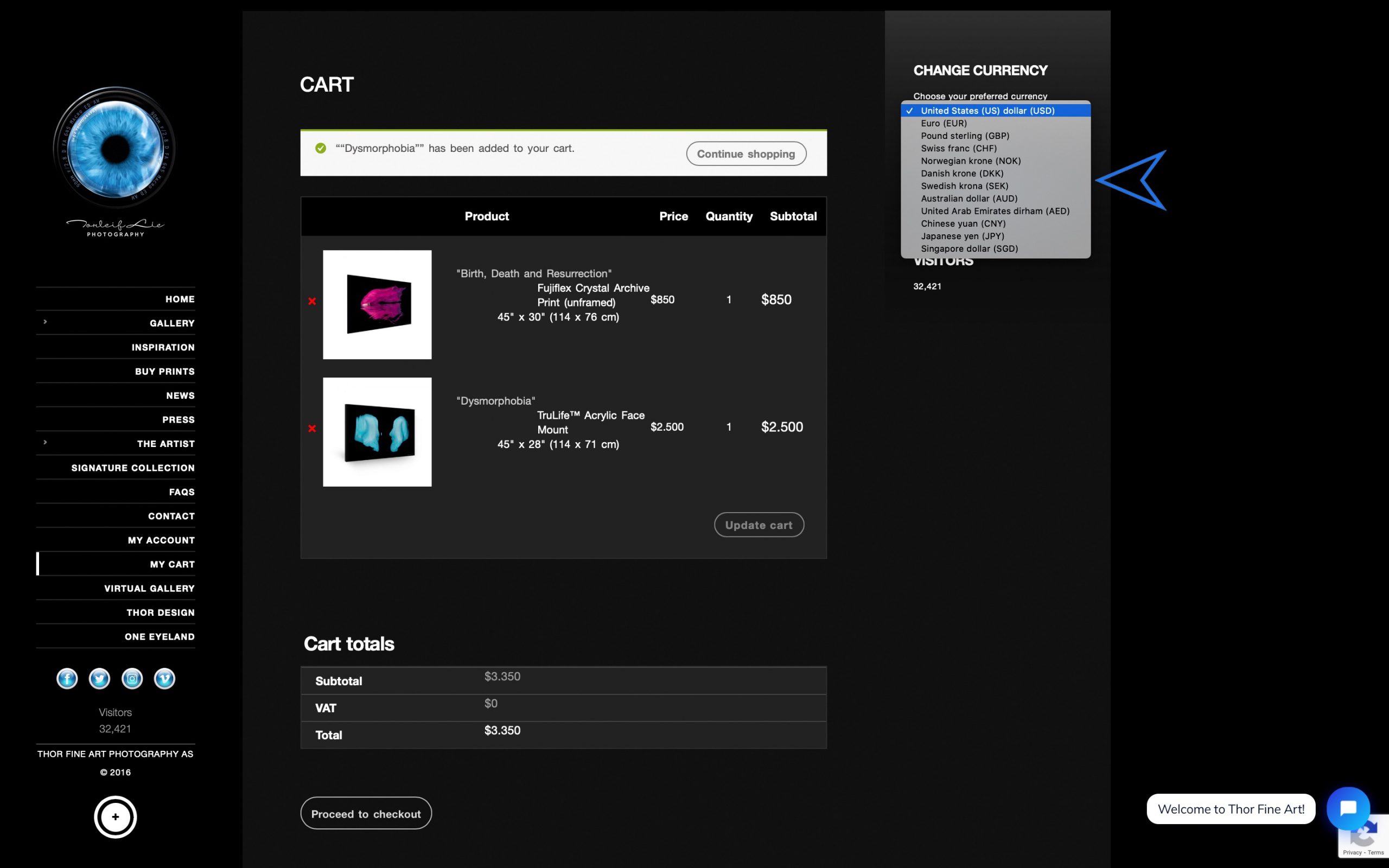A detailed, cleaned-up caption for the described image:

---

The image depicts a webpage with a black background, designed for an art gallery or online store. The left-hand side features a navigation menu with the options: Home, Gallery, Inspiration, Buy, Prints, News, Press, The Artist, Signature Collection, Contacts, My Cart, Virtual Gallery, Thor Design, and Island. In the upper left corner of this menu, there's a small image of a blue donut, beneath which is text too small to read.

The main content area of the page displays a shopping cart overview at the top, indicating a subtotal of $3,350 with no VAT tax applied. The cart contains two pieces of art: "Birth, Death, and Passion" listed at $850 with dimensions of 45 by 30 inches, and "Dysmorphia" priced at $2,500 and measuring 45 by 28 inches.